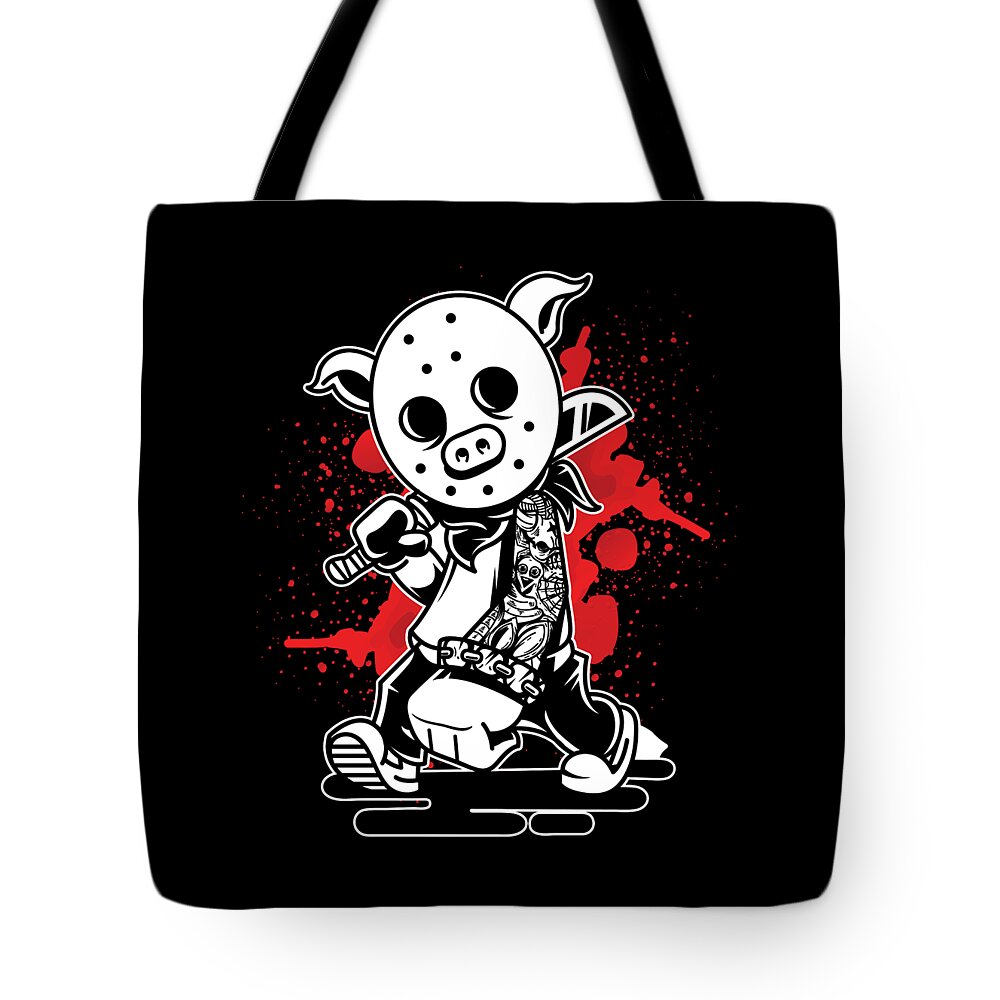This detailed photograph showcases a black rectangular tote bag, likely made of fabric or canvas, prominently displayed against a stark white background. The bag features a striking graphic of a menacing figure with an outlandish pig-like face mask complete with large, animal-like ears. The figure carries a large machete or saber casually draped over one shoulder and sports a white jacket adorned with a depiction of a dark-eyed, triangular-faced woman, possibly a vampire, on the sleeve. His ensemble is completed with black pants and sneakers. Surrounding the character is a dramatic splash of red, reminiscent of blood. The graphic exudes a dynamic, slasher cartoon feel, with tattoos and intricate designs possibly covering the character's arms or garments. The combination of these vivid and unsettling elements creates a compelling and edgy visual impact on the sleek, dark surface of the tote bag.